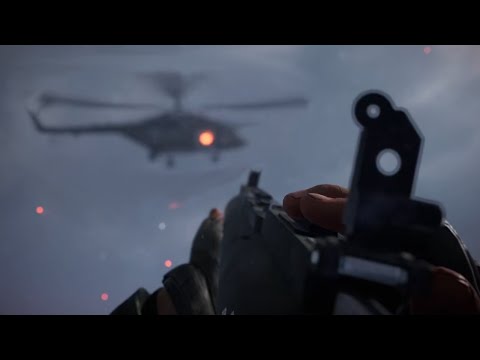This detailed image portrays a tense, nighttime scene juxtaposing foreground and background elements to create a vivid sense of action and perspective. In the foreground, viewed from a third-person point of view, there is an individual gripping a large, black automatic weapon. The person's gloved hands are in action; the left hand braces the bottom of the gun while the right hand manipulates something on the top. The gloves are fingerless, revealing parts of the fingers adding to the gritty realism of the scene. A viewfinder is prominently positioned in front of the person, aligning with their sightline toward the main focus in the distance.

In the background, a blurry attack helicopter looms amidst a dark, cloudy sky. The helicopter's rotors are whirling, indicated by their blurred appearance, and an orange light glows on the side of its body. The cabin of the helicopter is also illuminated, though it’s unclear if the light signifies a gun or is merely part of the cabin's interior lighting. Various red and white lights can be seen in the distance below the helicopter, adding depth to the night scene and hinting at either distant cityscape lights or other aerial vehicles. Black bars frame the top and bottom of the photograph, perhaps suggesting a cinematic or video game screenshot format. This dramatic composition captures the moment right before a potential action, blending the atmosphere of war with a striking visual narrative.